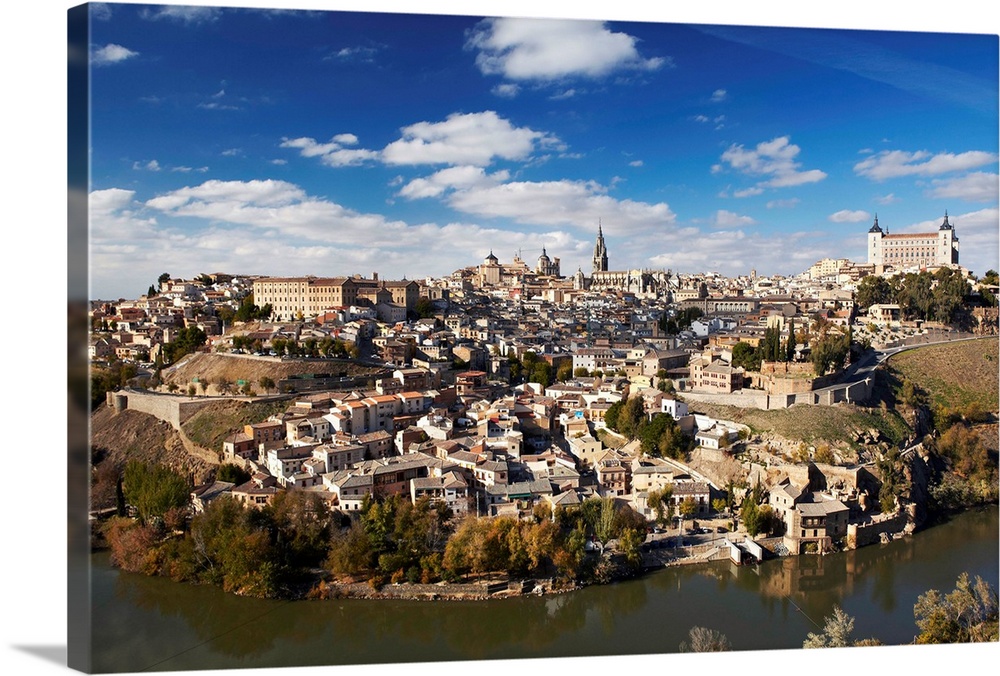The image showcases a picturesque neighborhood next to a dark, murky body of water, possibly a river, with a vibrant blue sky overhead sprinkled with fluffy white clouds. The scene unfolds on a bright, sunny day, suggesting a warm, summery atmosphere. On the banks of the water, interspersed with trees exhibiting a mix of green and autumnal hues of red and yellow, a series of charming two-story homes, resembling townhouses, begin to populate the landscape. The majority of these buildings are colored in white with brown accents, and they evoke an architectural style that hints at an early 1900s European influence. Further into the background, the cityscape ascends slightly uphill, where taller structures emerge, including a notably high building to the far right. There’s an indistinct yet recognizable structure at the center towards the back, adding an element of curiosity. To the left, more buildings rise, possibly indicating a blend of residential and business establishments, all contributing to the charm and historical feel of this serene small town.